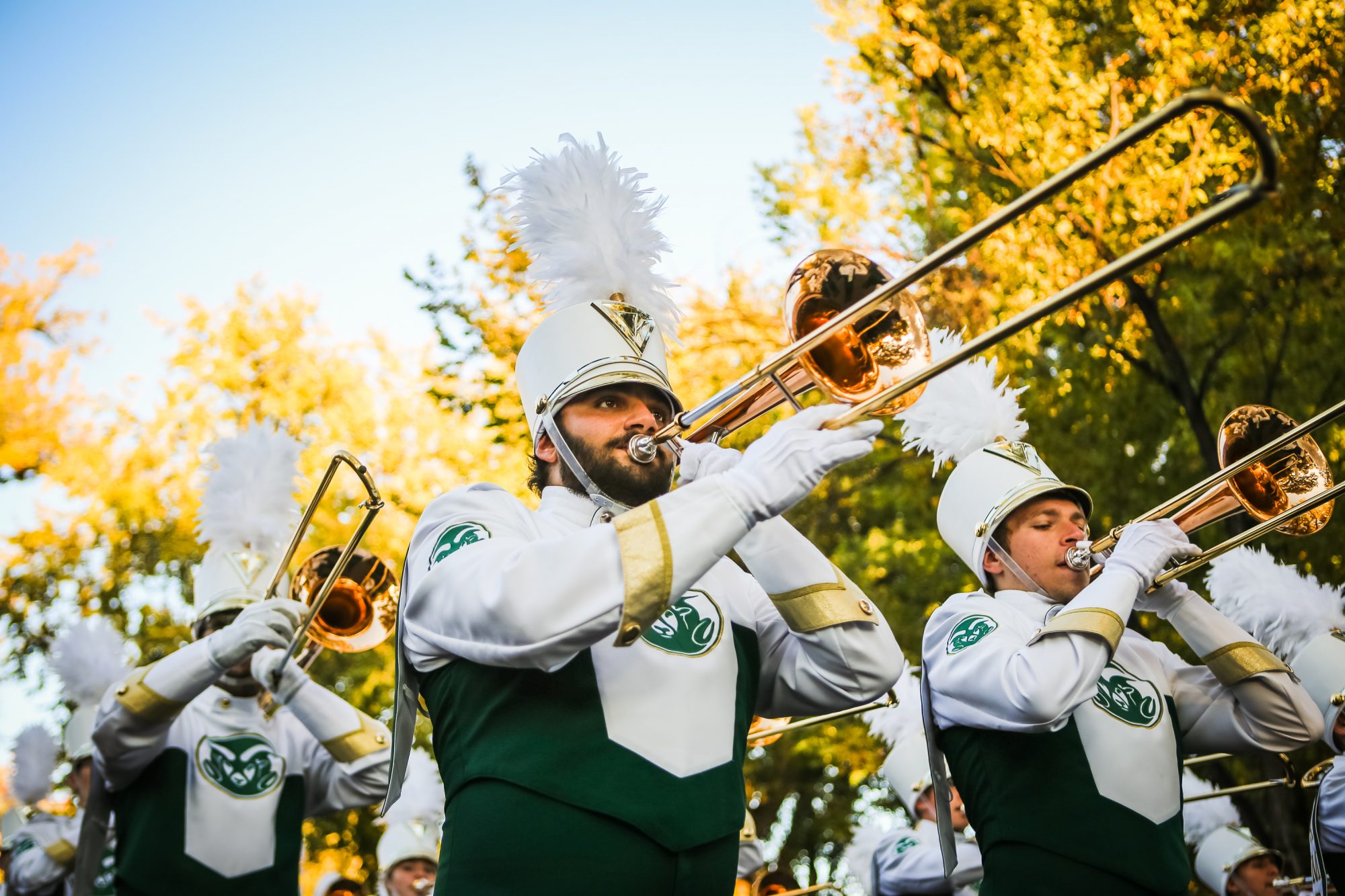This photograph captures a vibrant scene of a marching band set against a picturesque outdoor backdrop of trees and a brightly lit blue sky. In the foreground, three band members are prominently visible, each engrossed in playing the trombone. Their uniforms are distinctive, composed of green pants paired with shirts that feature white chest and sleeve areas adorned with intricate green designs. The ensemble is completed with white gloves trimmed with gold borders and striking white and gold hats crowned with elegant white feathers. Additional band members can be discerned in the background, contributing to the harmonious atmosphere of the image.